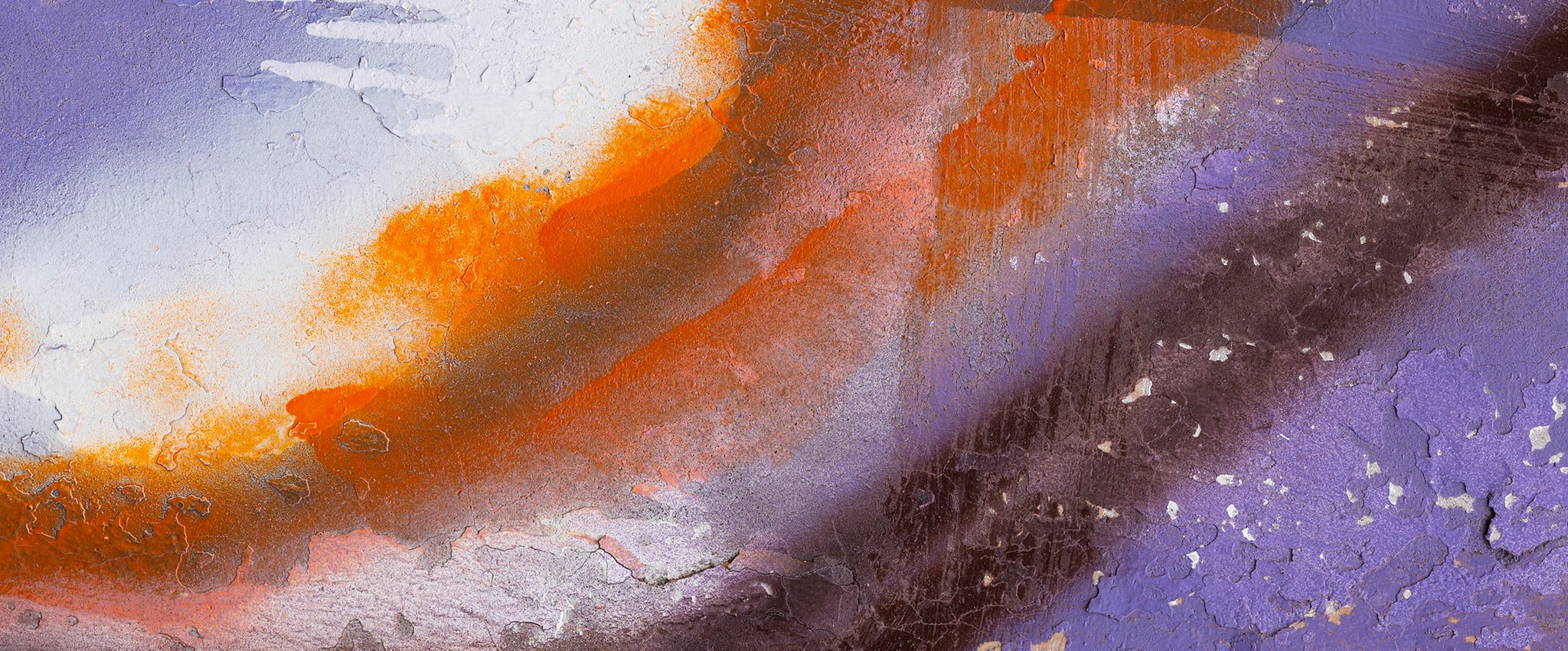This photo captures the side of a weathered adobe or textured clay wall, once adorned with a vibrant abstract mural. The mural, now deteriorating, features remnants of rich colors: a purple background with a dark purple stripe at the bottom right corner and an orange stripe parallel above it. The paint appears to have been spray-painted, evidenced by the streaks where the paint dripped. The once-lively artwork has faded, with the paint peeling and showing signs of age, giving the wall a neglected yet nostalgically artistic appearance.